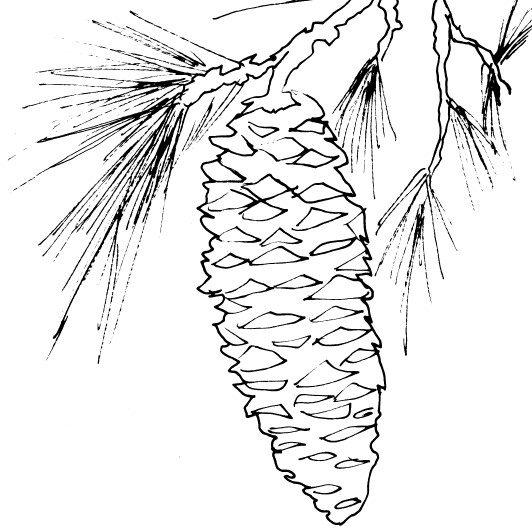This detailed black and white sketch features a single, scraggly pine cone prominently centered, measuring about four inches long. The pine cone exhibits an intricate array of grooves, ridges, and triangular jutting pieces, giving it a rough and sharp appearance. Small black lines speckle its surface, emphasizing its texture. The pine cone dangles from a branch adorned with clusters of pine needles. These needles, while spiky, appear less rough than the pine cone itself. Additional branches with more pine needle clusters extend to the left and right, filling the background with a natural, yet simple, composition reminiscent of a child's coloring book. The white background contrasts sharply with the dark, sketch-like quality of the branches, needles, and central pine cone.